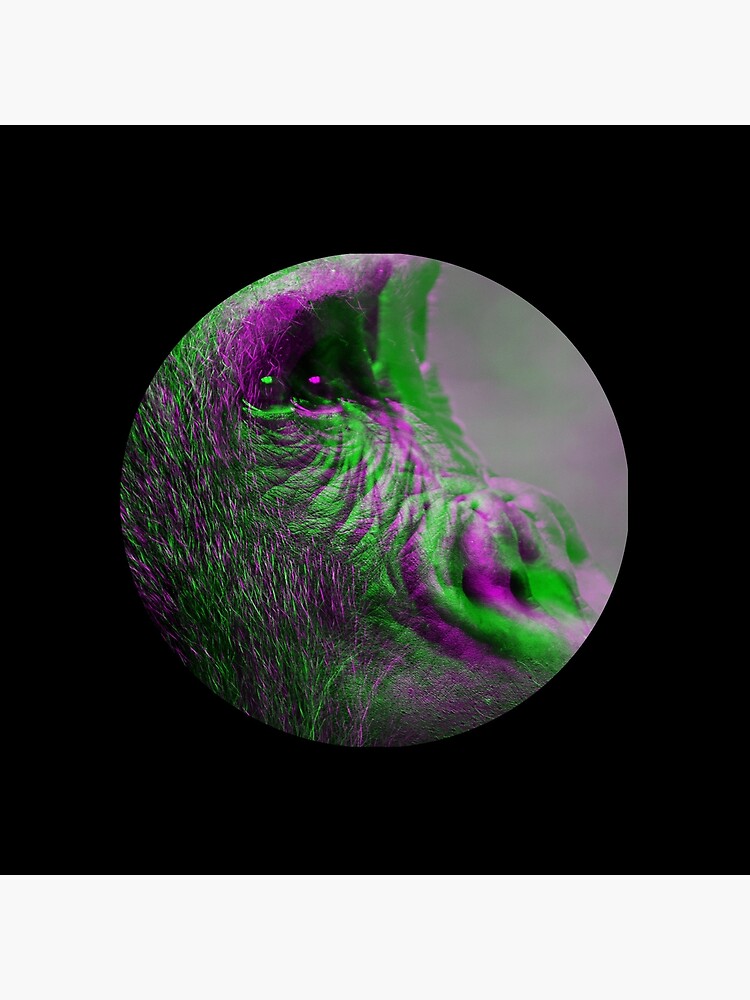The image is rectangular, measuring about 4 inches by 5 inches, featuring a solid black background. At the center, a circular cutout—approximately 2.5 inches in diameter—reveals a close-up of a gorilla's face, primarily focused on its right side profile. The gorilla's face, naturally dark with visible fur, has been manipulated to exhibit a chromatic aberration effect, resulting in overlapping, multi-toned, green and pink duplicates. This creates an impression of the face having multiple eyes and noses in a spider-like arrangement. The gorilla's eye is open, and it appears to be looking slightly upward towards the top right corner. The image inside the circle is set against a mostly light gray background, while the rest of the picture remains plain with a light gray header along the top edge.